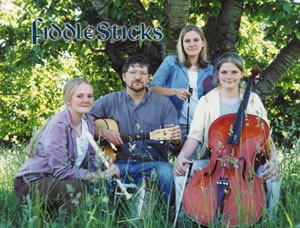In this small horizontal rectangular photograph titled "Fiddlesticks" in green text with a white border in the top left corner, a casual and cozy outdoor setting features a band, possibly a family or local group, gathered under a sprawling tree with abundant green leaves. The lush, tall grass reaches up around them, partially obscuring some details and giving a grounded, natural vibe.

From left to right, the band comprises: a woman crouching in brown pants, a white shirt, and a purple long-sleeve button-up top, holding a white flute loosely in her right hand; a man seated on a chair, clad in blue jeans and a gray buttoned long-sleeve shirt, with glasses on his face and a light brown acoustic guitar resting in his lap; behind him stands a woman, visible from the waist up, dressed in a denim jacket with rolled-up sleeves and a white shirt underneath, her hand gripping what seems to be a fiddle; and on the far right, another woman dressed in something white is proudly holding a huge bass.

The setting, combined with their relaxed attire and the various musical instruments, evokes a charming and tight-knit atmosphere, hinting at an intimate performance or promotional image for this endearing group. Their casual demeanor and the rustic backdrop of the tree and grass contribute significantly to the photograph's warm, inviting feel.